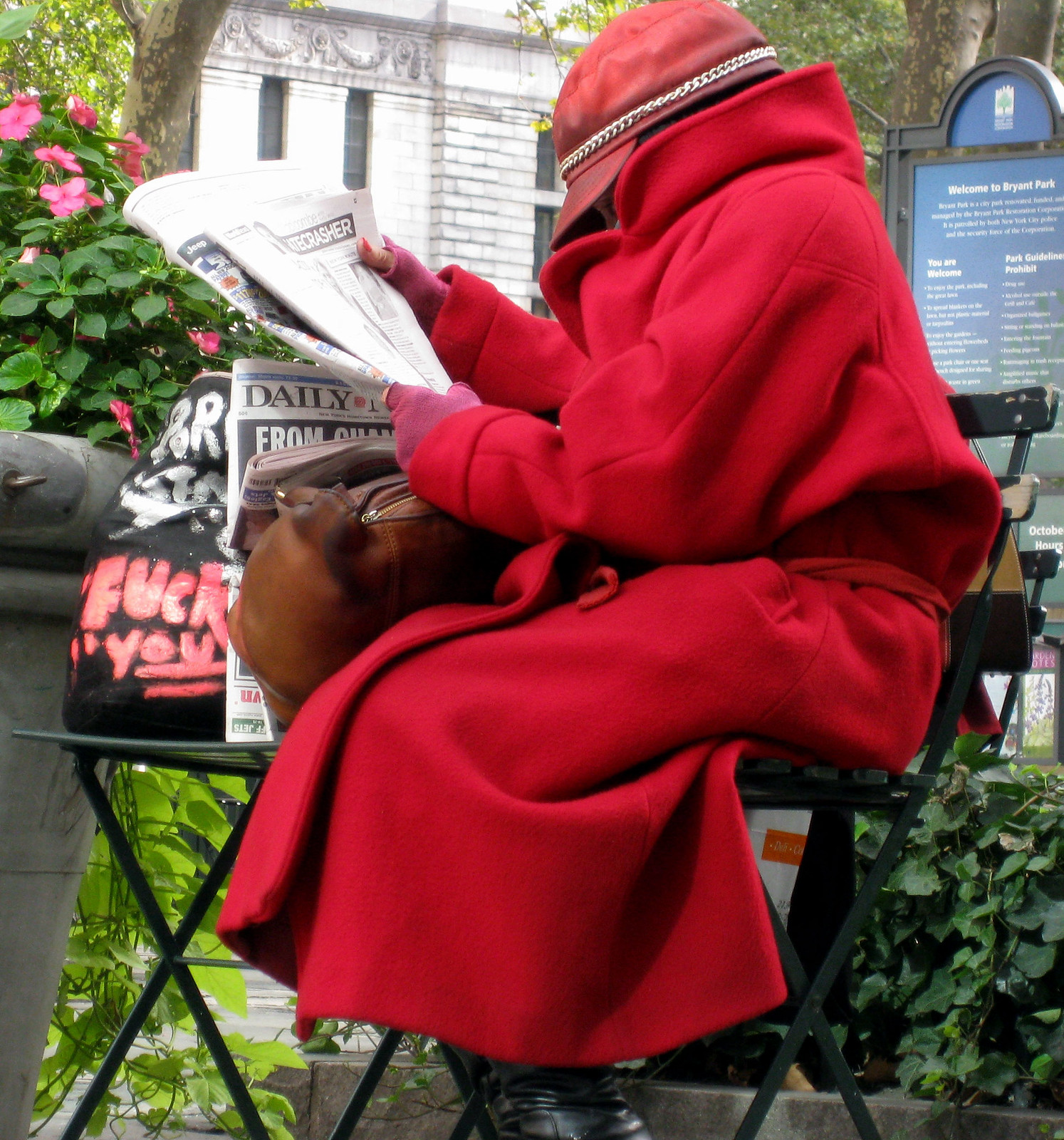In this outdoor photograph, a person, likely female, is sitting scrunched up on a park bench in what appears to be Bryant Park in New York City. She wears a striking ensemble consisting of a long red coat that reaches down to her calves and has a collar pulled up high, obscuring most of her face except for a glimpse of the bridge of her nose. She also dons a red short-billed hat adorned with a chain, and pink fingerless gloves revealing red-painted fingernails. She is intently reading the Daily Mail newspaper.

Resting in her lap is a brown purse, while a separate black bag with bold red text reading "FUCK YOU" and additional white writing sits on the chair next to her. The bench itself is black, and the surrounding scene includes elements characteristic of a New York City park: a lush backdrop of greenery, some rose bushes with pink flowers, and a white-faced stone building in the background. Additionally, there is visible signage that reads "Welcome to Bryant Park," and a blue sign and a pot further enrich the setting. The ambiance is a mixture of urban elements and serene park scenery.